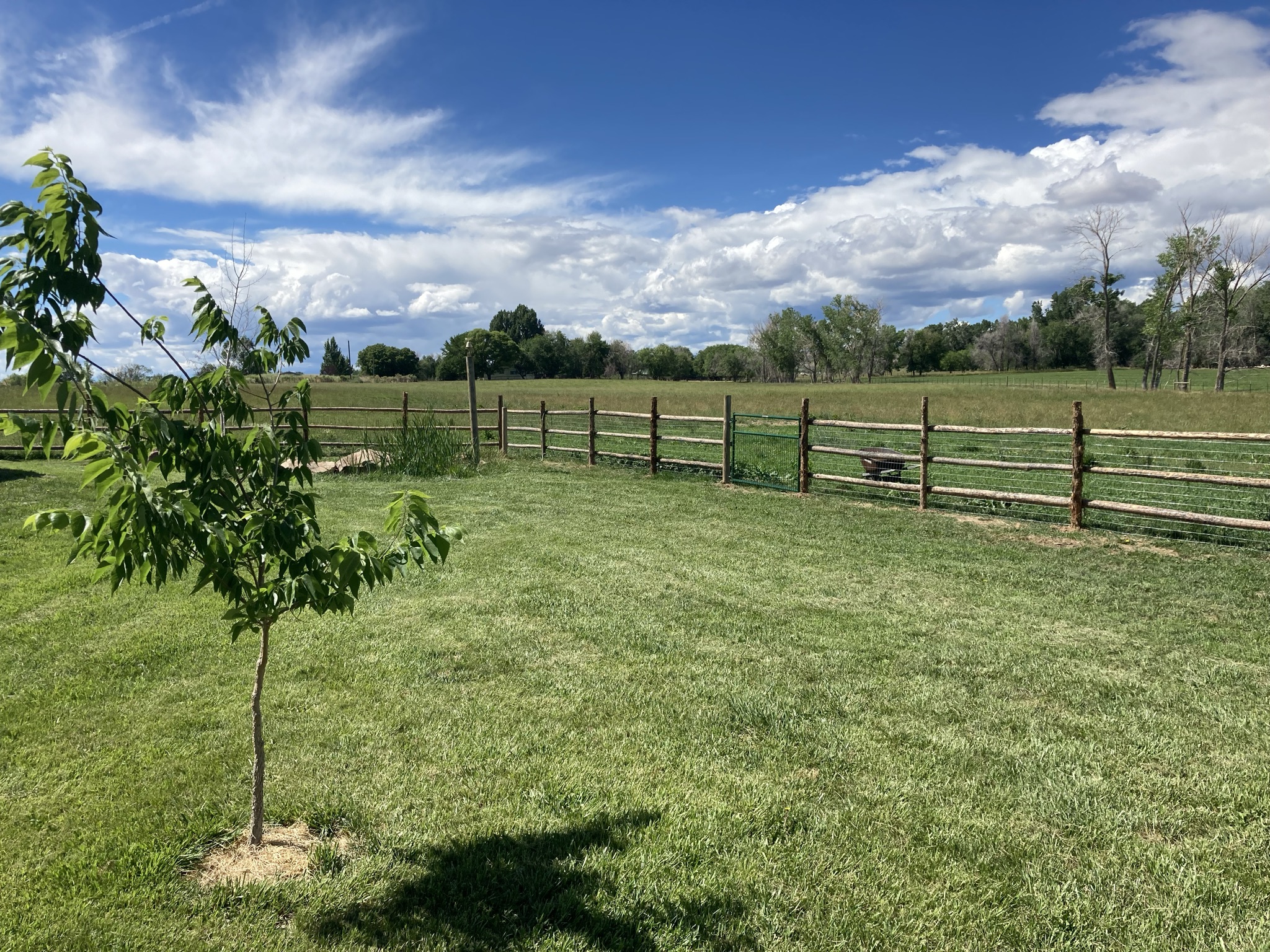In this vibrant landscape photograph, taken under a clear blue sky dotted with puffy white clouds, the primary focus is a small, recently planted tree situated in the foreground. The scene, captured on a sunny midday in what appears to be either spring or summer, reveals detailed shadows indicating the bright, early afternoon sun. The tree stands in the center of a neatly manicured, lush green pasture, which is enclosed by a handmade wooden fence reinforced with chicken wire. The fence stretches from the right side of the photograph, forming a corner in the middle, and extends across to the left. Just inside this fence is a small rock formation and a post with a bell. A gate in the fence opens out into a larger field with slightly taller grass. In the distance, a diverse tree line marks the horizon, suggesting a rural setting full of natural beauty. There are no animals within the scene, which emphasizes the serene and tranquil atmosphere of the landscape.